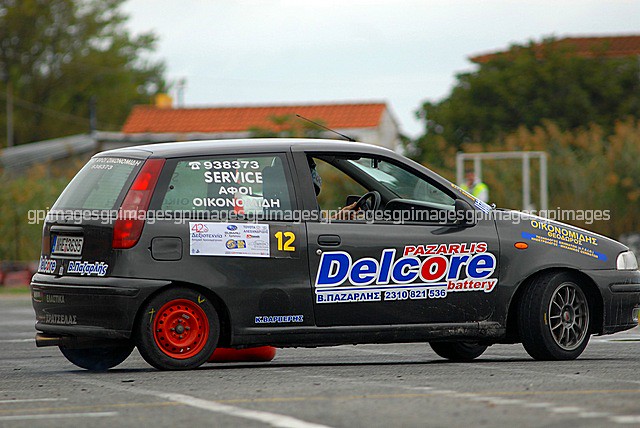In the foreground of this wide rectangular image, a small, black, four-seater car is prominently featured, facing to the right. The car's passenger side, which faces the camera, is adorned with blue and red lettering that reads "Pazarlis Delcor Battery," suggesting it might be battery-powered. A number "12" is also visible on the side. The back window displays a telephone number, "938-373," along with the word "service" and some additional, unidentified text.

The car is parked on a gray parking lot, marked with white and yellow lines. Notable is the red-metal rim on the back wheel, which could indicate a spare tire. Above and around the car, the background reveals a white house with an orange or red roof and patches of green forest on either side. The overcast sky looms above, adding to the subdued atmosphere.

Blurred and small, a person wearing a yellow construction jacket can be seen behind the hood of the car, adding a hint of human presence. Additionally, a watermark reading "GP images" is repeatedly stamped across the center of the picture.